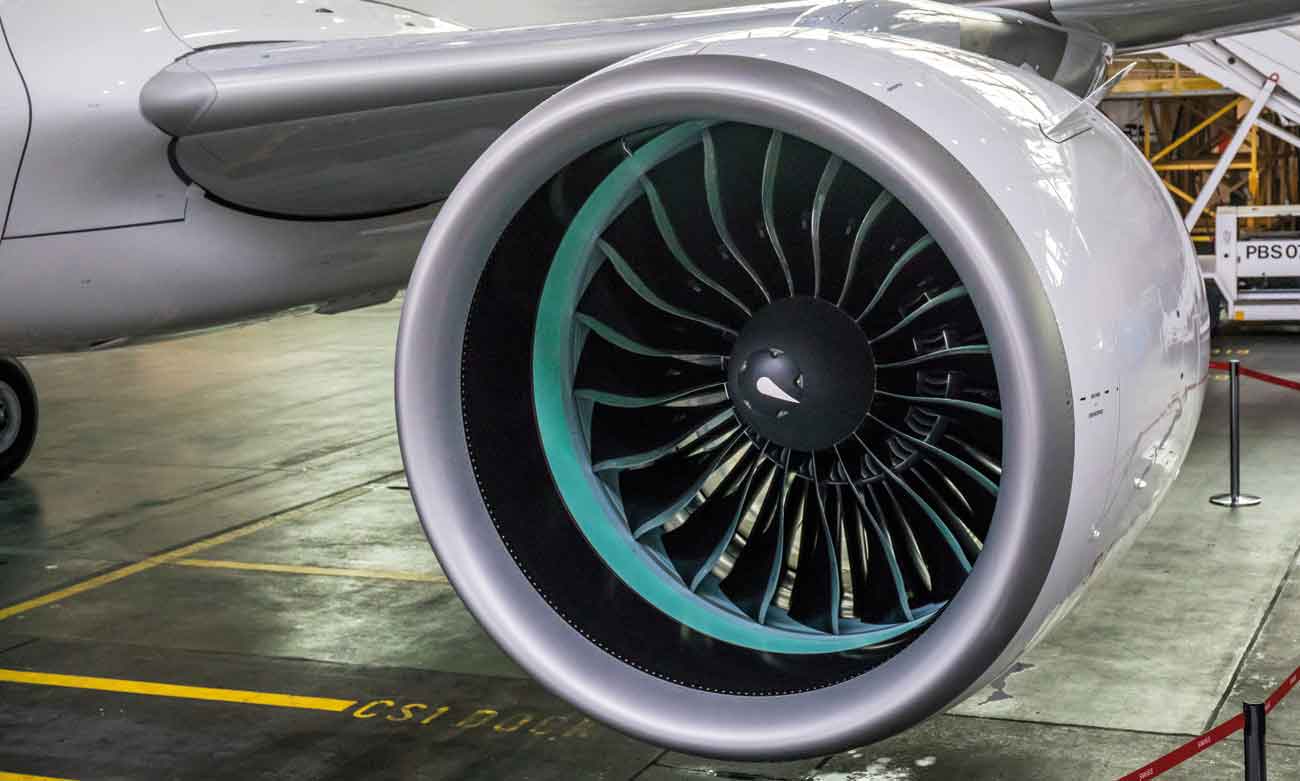The photograph captures a detailed view of an airplane engine, specifically focusing on the inside of the turbine. The engine, primarily white with a glossy metallic finish, features a silver steel brim encasing it. Within the cylinder, the turbine blades form a circular pattern, highlighted by a distinctive teal color against a predominantly black interior. Extending from the right-hand side to the left side of the image, the wing of the plane, also glossy white, is visible, attaching seamlessly to the plane's base. The aircraft rests on a cement floor marked with yellow lines and labeled "CS-1 dock," with additional red security pathway markings on the right. A yellow scaffold and some background activity hint at a hangar setting, suggesting the plane is parked indoors.